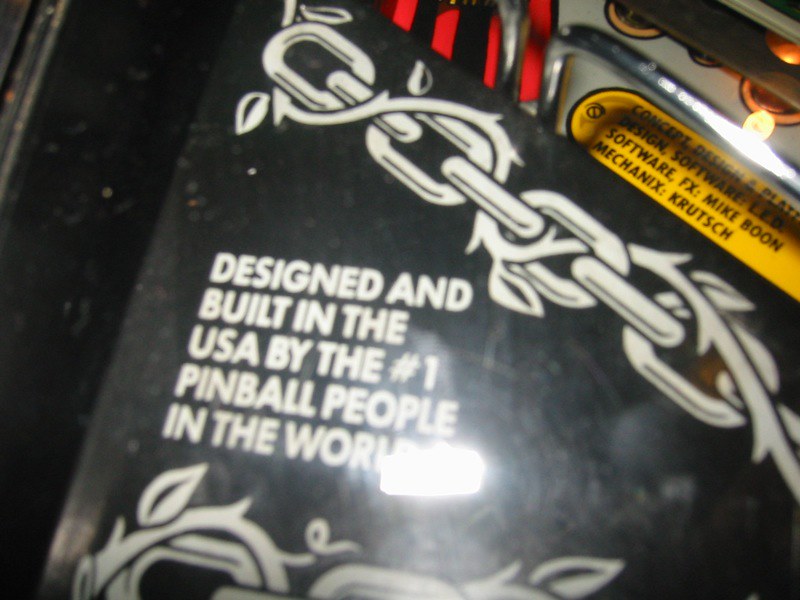This image features a close-up view of a pinball machine panel, predominantly set against a black background. Prominent white text at the center proudly declares, "Designed and Built in the USA by the Number One Pinball People in the World." This text is framed above and below by an elaborate white chain design intertwined with delicate ivy, adding a touch of classic elegance. 

Above this central message, a bright yellow label lists various contributions to the machine's creation: "Concept Design and Play Design Software Led Software FX: Mike Boone, Mechanics: Nix Krutsch." Above this label, red and black stripes add a striking, bold accent.

On the right-hand side of the image, a white segment hints at the edge of the pinball machine, with what appears to be a pinball light in the upper right corner. Due to the close-up nature of the photo, the exact part of the machine is indeterminate, but it vividly captures the meticulous and ornate craftsmanship of the design.